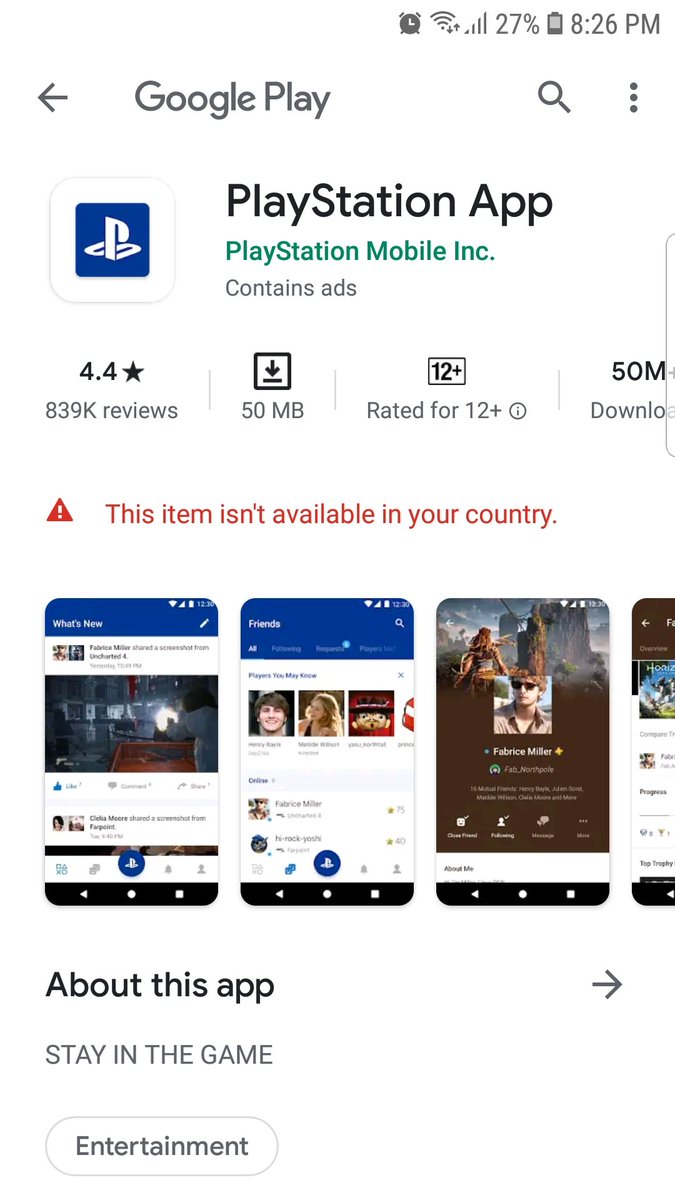The screen capture showcases the Google Play Store interface at 8:26 PM, with the battery at 27%, full cell service bars, an active Wi-Fi connection, and an alarm clock icon in the status bar. At the top of the screen, a back arrow, the "Google Play" title, a search icon, and a three-dot menu are visible on the banner. 

The main focus is on the "PlayStation App" by PlayStation Mobile Inc., which contains ads. The app has a PlayStation logo next to the title. It boasts a 4.4-star rating from 839,000 reviews, a download size of 50 MB, a 12+ age rating, and over 50 million downloads. An orange warning triangle indicates that "This item isn't available in your country."

Following this notification, there are three full and one partial screenshots of the app in use. Further down, the "About this app" section is indicated with a right-pointing arrow. The description reads "Stay in the game," next to an entertainment category icon.